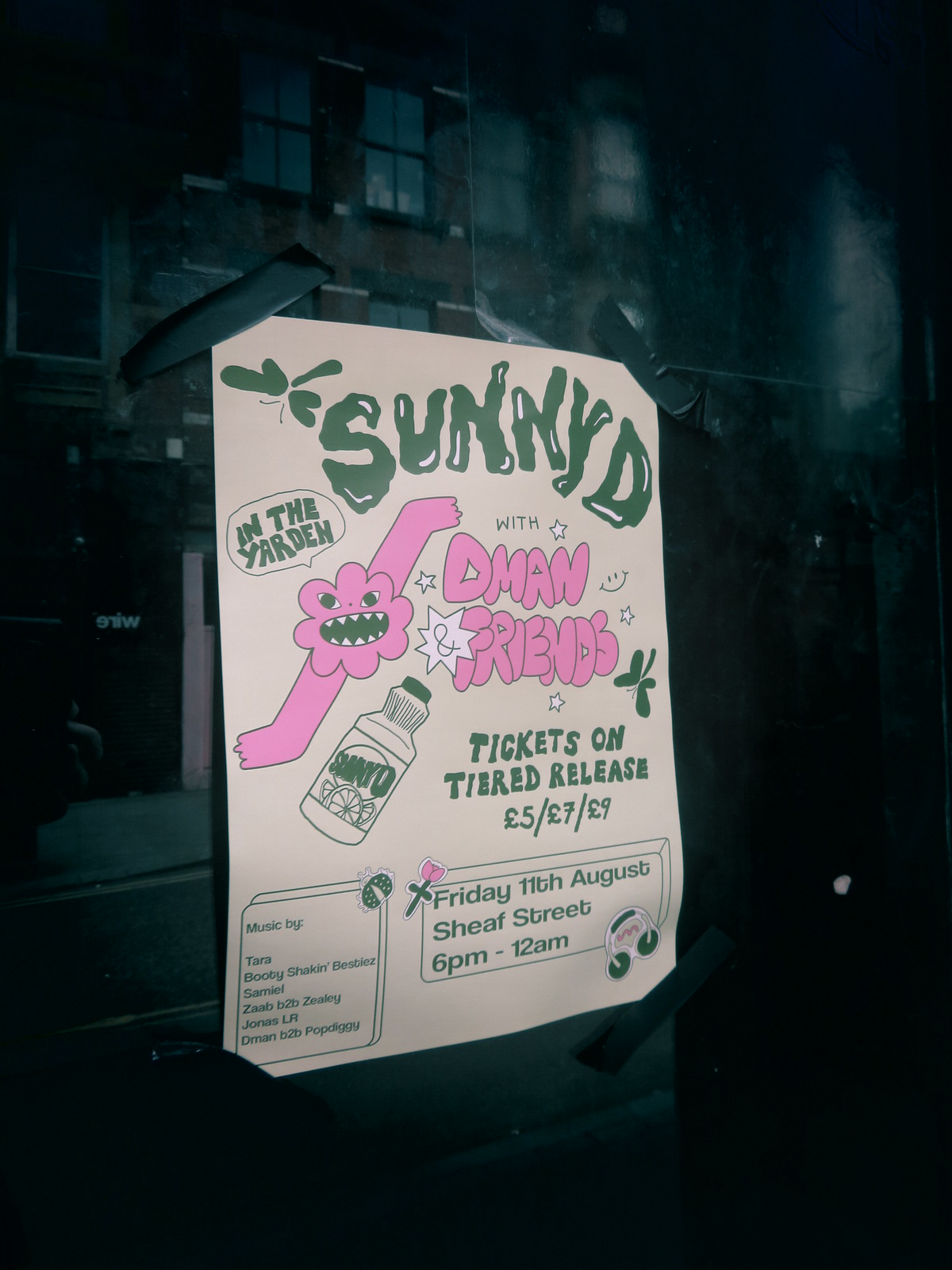This photograph captures a glossy surface, either a window or wall, reflecting an adjacent brick building with multiple black-framed windows, a sidewalk, and a street. The focal point is a rectangular poster, taped at all corners with black tape, on off-pink paper. The top of the poster features the text "Sunny D" in greenish-black, stylish block letters. Below, in a speech bubble, are the words "In the Garden," accompanied by a pink cartoon cloud with a face and stretched-out arms. Next to it, in pink letters, reads "D-Man Friends." The poster includes a drawing of a Sunny D bottle and is detailed with event information: "Tickets on tiered release £5/£7/£9, Friday 11th August, Sheaf Street, 6pm-12am." Additional details note music by Tara, Booty Shakin' Bebe's, Samuel, Zarb B2B Zealy, Jonas LR, D-Man, and B2B Pop Diggy.